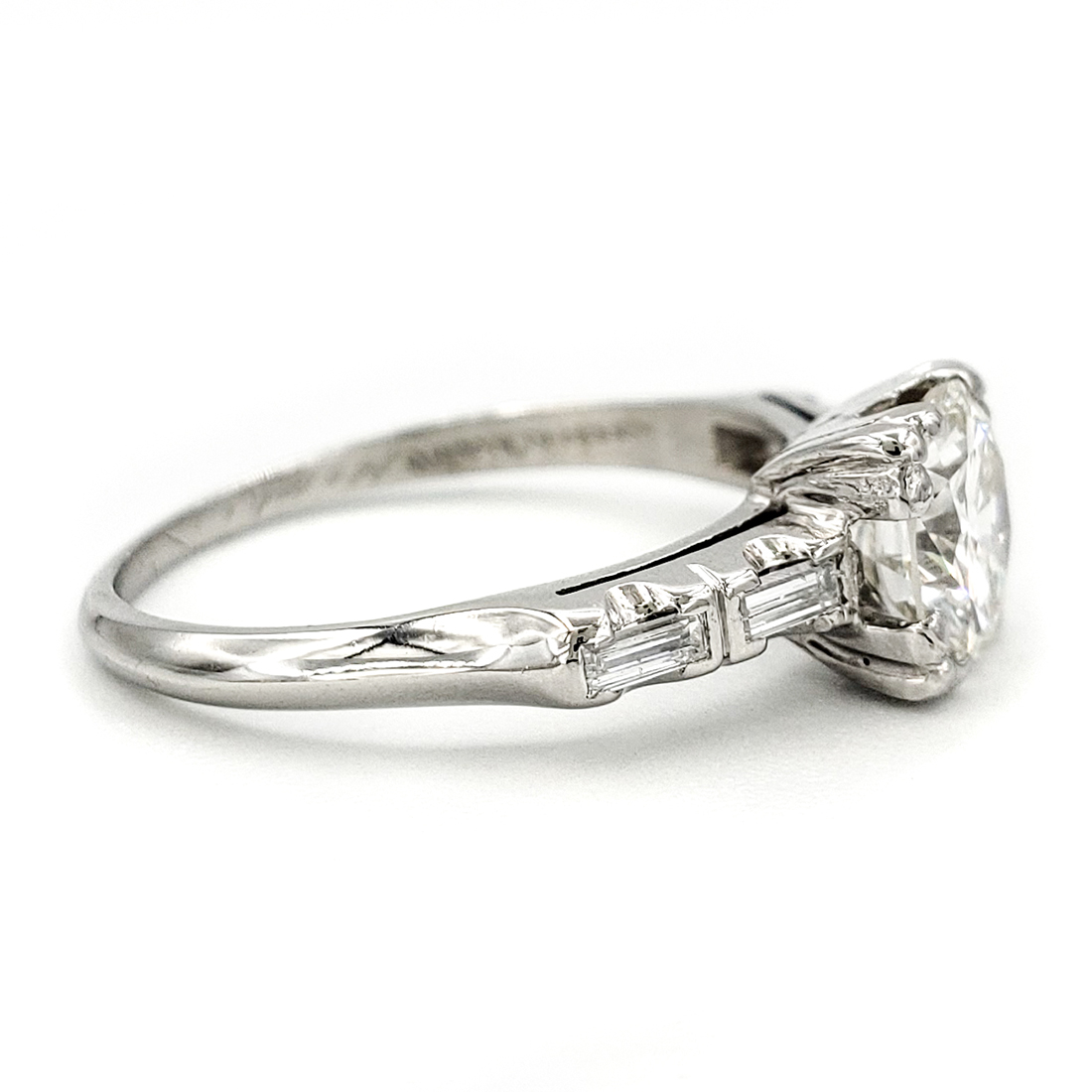This detailed image features a close-up view of an engagement ring set against a white background. The silver, white gold, or platinum band, which is smooth and subtly dips in places, encircles the large, notable center diamond. The diamond, which could be either round or princess cut, faces towards the right, while the bottom of the band is to the left, displaying a side view of the ring. Flanked on either side of the central diamond are two smaller horizontal stones, likely baguette or emerald cut. In the image, these stones on the opposite side are obscured by the main diamond. Despite lacking a glittering brilliance, the ring emanates a low-key shine. Inside the band, there is an engraving or marking, although the blurriness of the photo renders it illegible. This engraving could either be decorative or indicative of the ring's usage.